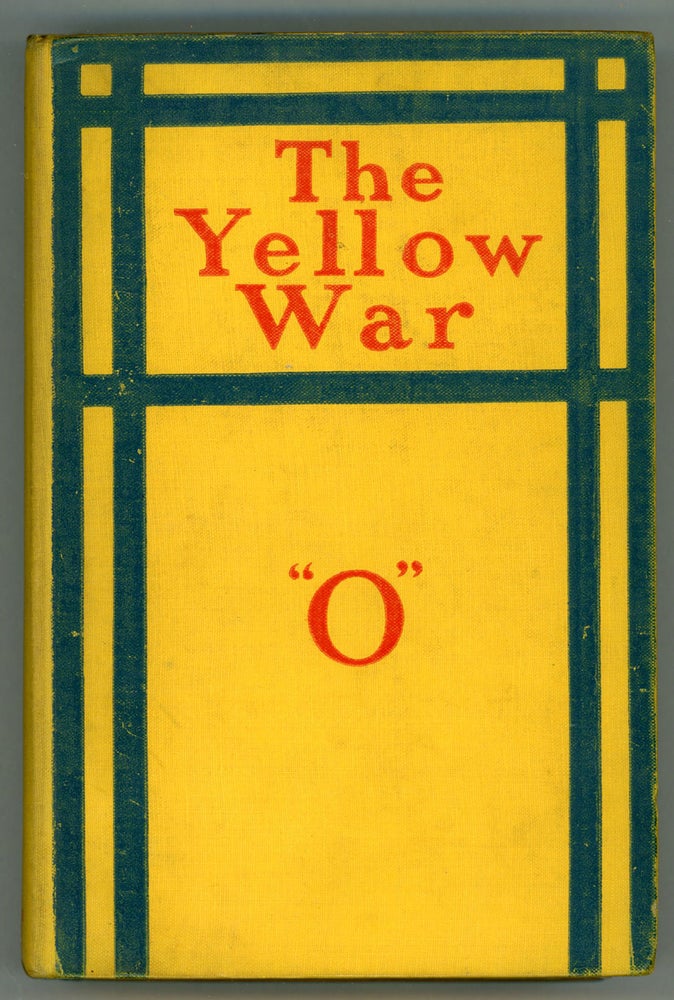The image depicts the front cover of an old, yellow book positioned on a light blue surface. The cover looks worn and tattered, with a vintage feel, likely from its simple glued binding. Prominently at the top of the cover, the title "The Yellow War" is written in bold red text, stacked vertically. This title is encased within a thick blue border, which is thicker than the font itself. Above and below this main title, additional blue lines run horizontally, with two vertical blue stripes framing the sides of the cover. In the lower portion of the cover, below the main title and its accompanying lines, the letter "O" in red, uppercase, and enclosed in quotation marks, is placed centrally. The cover, through its minimalist yet striking design, invokes a sense of antiquity and intrigue.